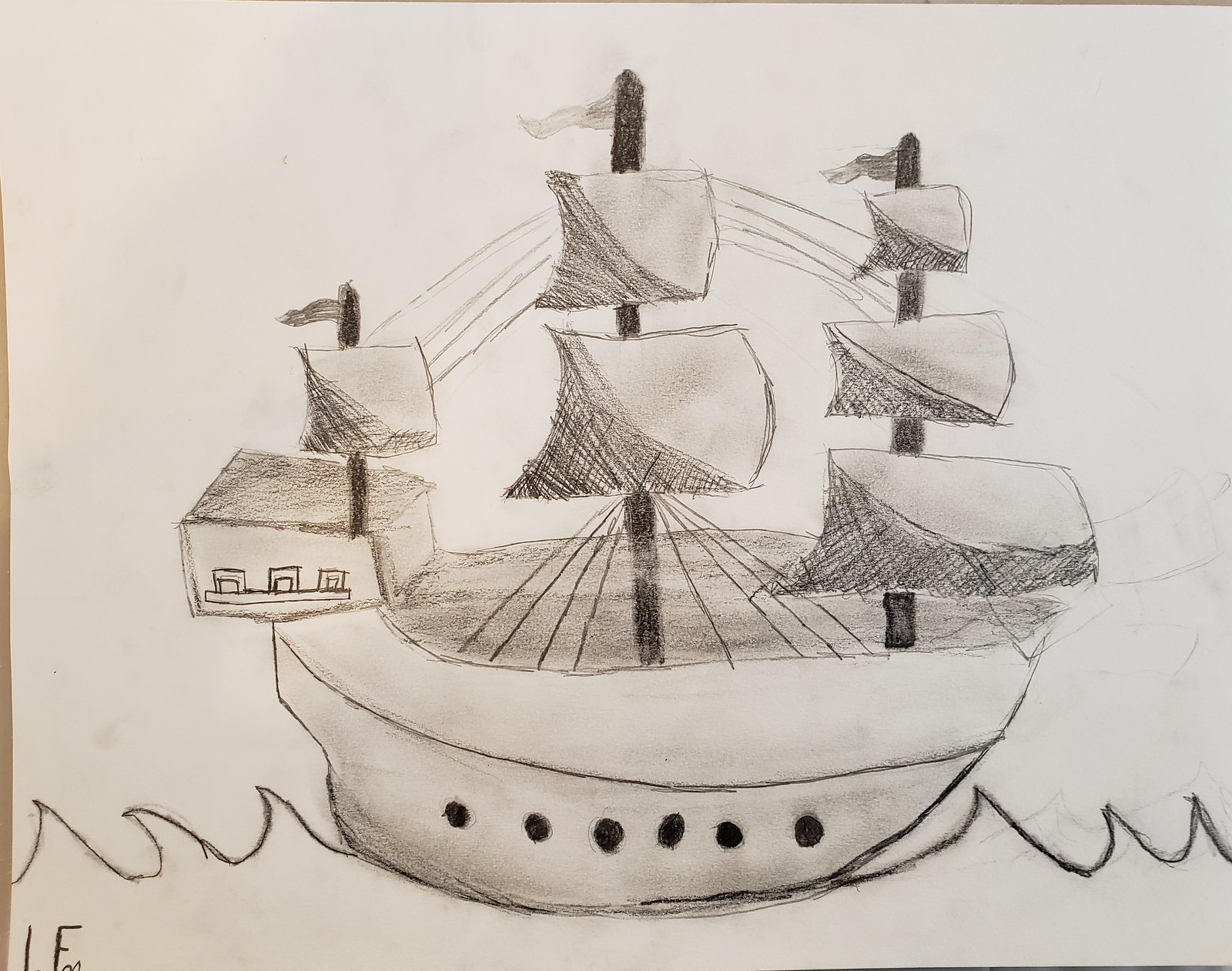This drawing, crafted in black pencil on white paper, showcases intricate, bold line work mimicking the turbulent waves of the ocean. The waves are characterized by sharp, peaked crests that curl downwards in a repetitive, rhythmic pattern. Amidst these dynamic waves sails a formidable, pirate-style ship. The vessel exhibits a semicircular hull with a flat base, crowned by an upper cabin that likely serves as the captain's quarters. The ship is equipped with three masts: the smallest mast at the rear with a single sail, the tallest central mast with two sails, and the forward mast, intermediate in height, adorned with three sails. The composition masterfully captures the essence of maritime adventure and the relentless energy of the sea.